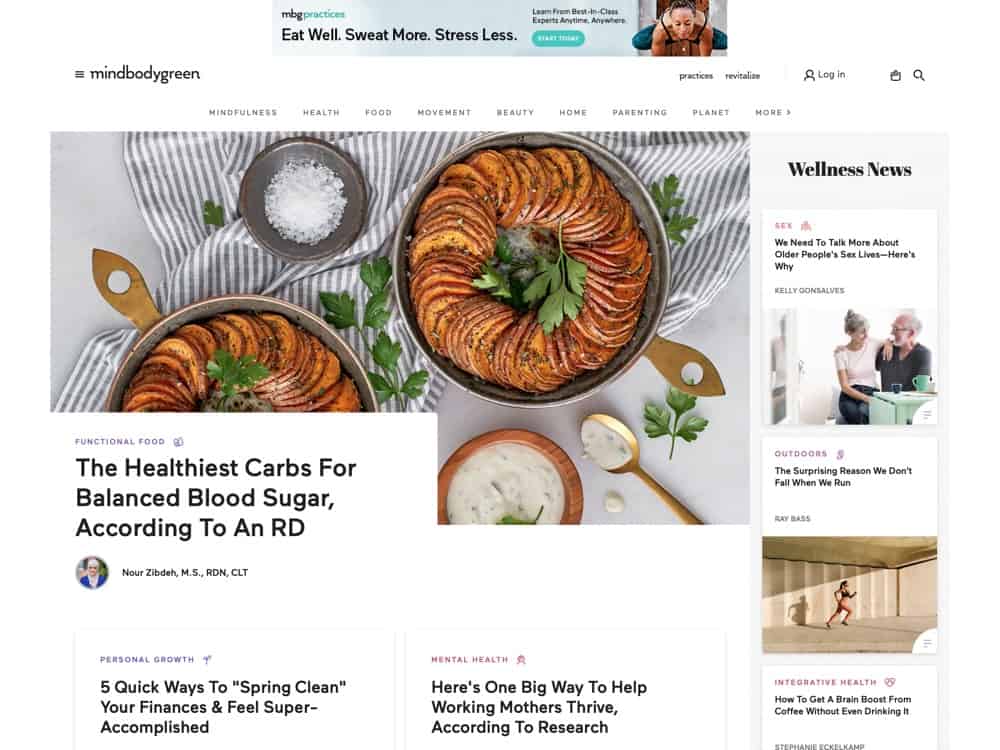**Descriptive Caption:**

The screenshot highlights a page from the MindBodyGreen website, a reputed hub for wellness content. In the top left corner, the MindBodyGreen logo is prominently displayed along with a three-lined menu icon. At the top middle, there's an engaging advertisement featuring a woman performing yoga, with the slogan, "Eat well, sweat more, stress less." The ad encourages users to "learn from best-in-class experts anytime, everywhere," accompanied by a clickable button.

Just below, the site’s extensive menu bar provides various options including Mindfulness, Health, Food, Movement, Beauty, Home, Parenting, Planet, and more. To the top right, additional menu options include Practices, Revitalize, and user account functionalities like logging in, with a shopping cart icon and search icon placed at the far right.

Dominating the central part of the image is a feature article titled "The Healthiest Carbs for Balanced Blood Sugar, According to an RD," authored by Noor Zipteh, MS, RD, CLT. The article falls under the category of Functional Food. The background image shows two dishes filled with what appears to be thinly sliced potatoes or vegetables, accompanied by a bowl of salt and a bowl of sauce, adding a visual flavor to the subject matter.

On the far right, the page includes a 'Wellness News' sidebar featuring various other articles, along with two more articles on different subjects towards the bottom of the page.